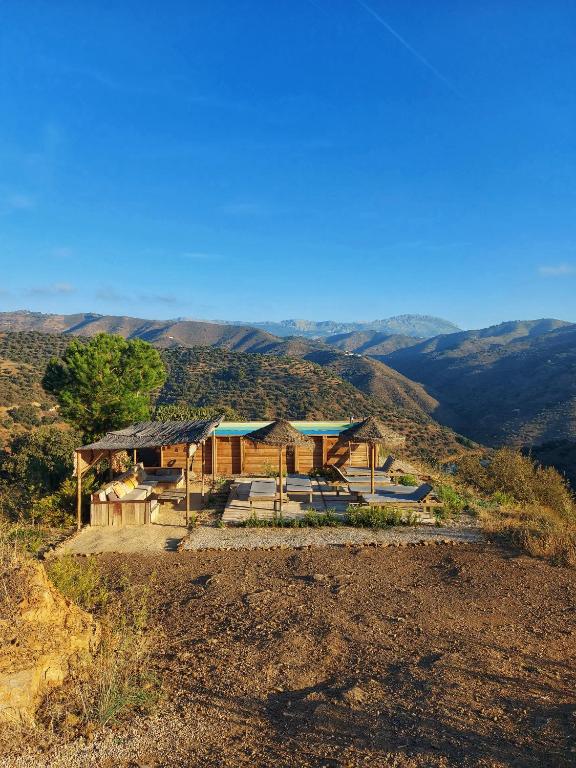This detailed landscape photograph, oriented in portrait, captures a striking scene of an arid mountain range under a crystal-clear blue sky with a hazy sun glow. In the foreground, on a flat, brown ground, sits a small wooden cabin that seems incongruously placed on this barren hillside. The cabin, evocative of a Hawaiian style, features a patio area adorned with tiki-style thatched umbrellas providing shade over cushioned wooden couches and beach chairs. The seating area, designed for comfort, includes two inclined beach chairs topped with wide thatched umbrellas, and another pair of vertical beach chairs with matching umbrellas. This intimate square courtyard also hints at an outdoor kitchen or seating area covered by a canopy made of round sticks. Nearby, a few short, scattered trees attempt to bring some verdant life to the otherwise dry setting. In the background, the rugged, barren mountains stretch out, enveloping the scene in natural grandeur while a cozy shelter offers a striking contrast to the surrounding wilderness.